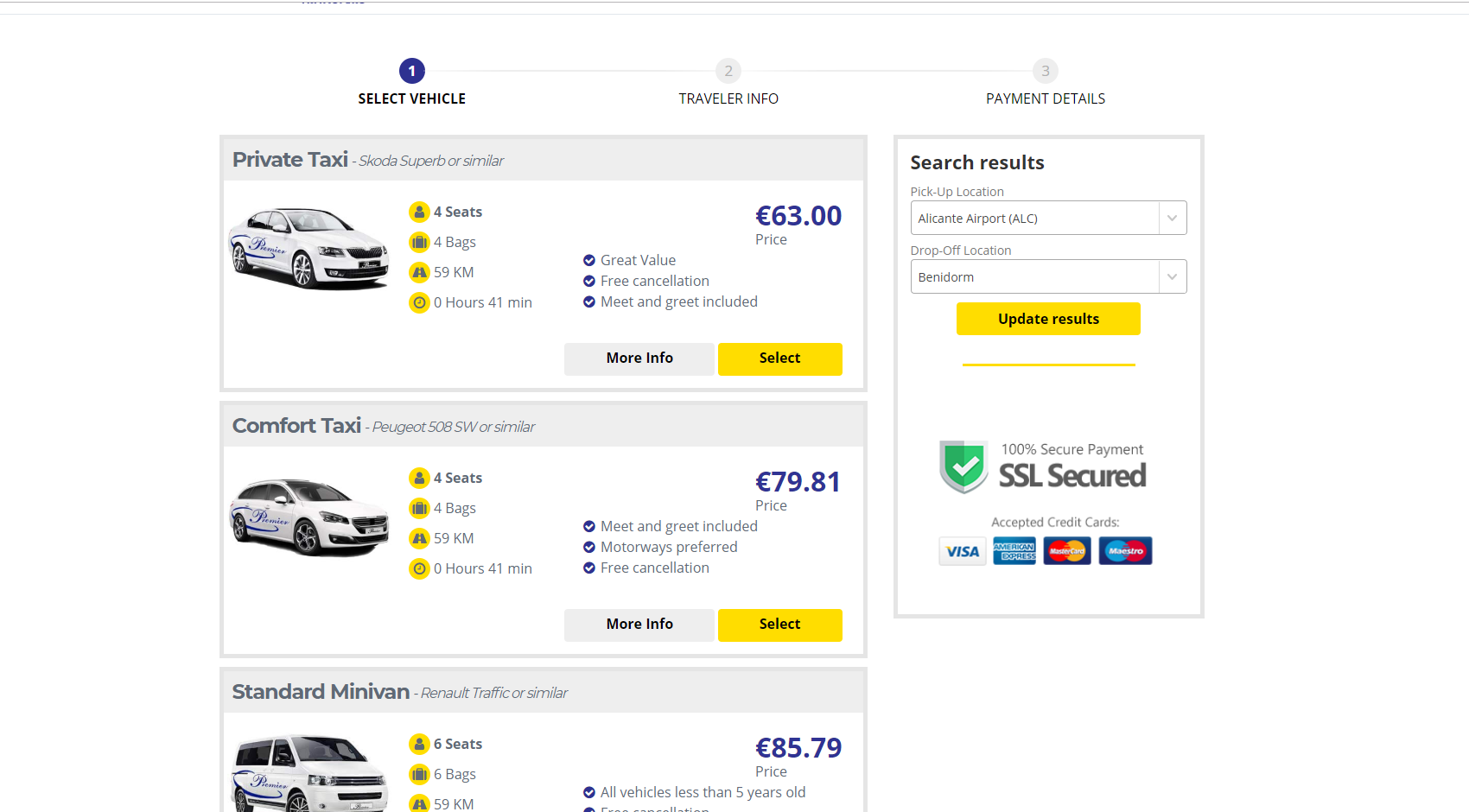**Screenshot of Car Rental/Taxis Selection Page**

At the top of the page, a progress bar labeled with three steps guides the user through the booking process: "1. Select Vehicle," "2. Travel Info," and "3. Payment Details." Below the progress bar, three rectangular vehicle options are presented:

1. **Private Taxi:**
   - **Details:** 4 seats, 4 bags, 59 km, 0 hours 41 minutes.
   - **Additional Features:** Great value, free cancellation, meet-and-greet included.
   - **Buttons:** A gray "More Information" button and a yellow "Select" button.
   - **Price:** $63.

2. **Comfort Taxi:**
   - **Details:** 4 seats, 4 bags, 59 km, 0 hours 41 minutes.
   - **Additional Features:** Meet-and-greet included, motorways preferred, free cancellation.
   - **Price:** $79.81.

3. **Standard Minivan:** 
   - **Details:** 6 seats, 6 bags, 59 km.
   - **Additional Features:** All vehicles less than five years old.
   - **Price:** $85.79 (partially cut off).

On the right side of the page, there is a sidebar with several supportive sections labeled "Search Results," "Update Results," and features SSL secured payment icons for Visa, American Express, MasterCard, and Maestro.